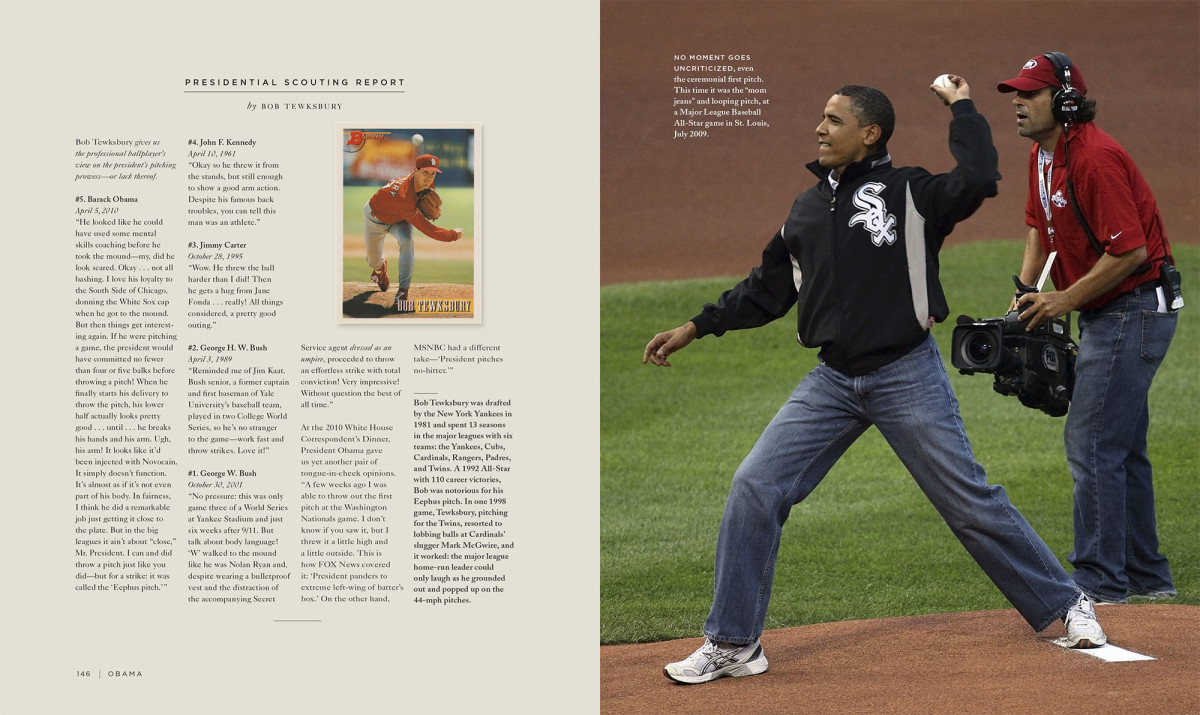The image displays a two-page spread from a baseball magazine. The left page, titled "Presidential Scouting Report" by Bob Tewberry, features an article too small to read clearly and showcases a trading card with a red logo that resembles "JJ," alongside a baseball player poised mid-throw. At the bottom of the left page, the word "Obama" and what appears to be a page number are visible. The right page presents a vivid photograph of President Barack Obama throwing a ceremonial first pitch at a baseball game. He is wearing a black Chicago White Sox jacket with white detailing from the shoulders to the waist, blue jeans, and white sneakers. His arm is pulled back, ready to throw the ball. Behind him stands a cameraman dressed in a red hat, red shirt, blue jeans, and headphones, capturing the historic moment.